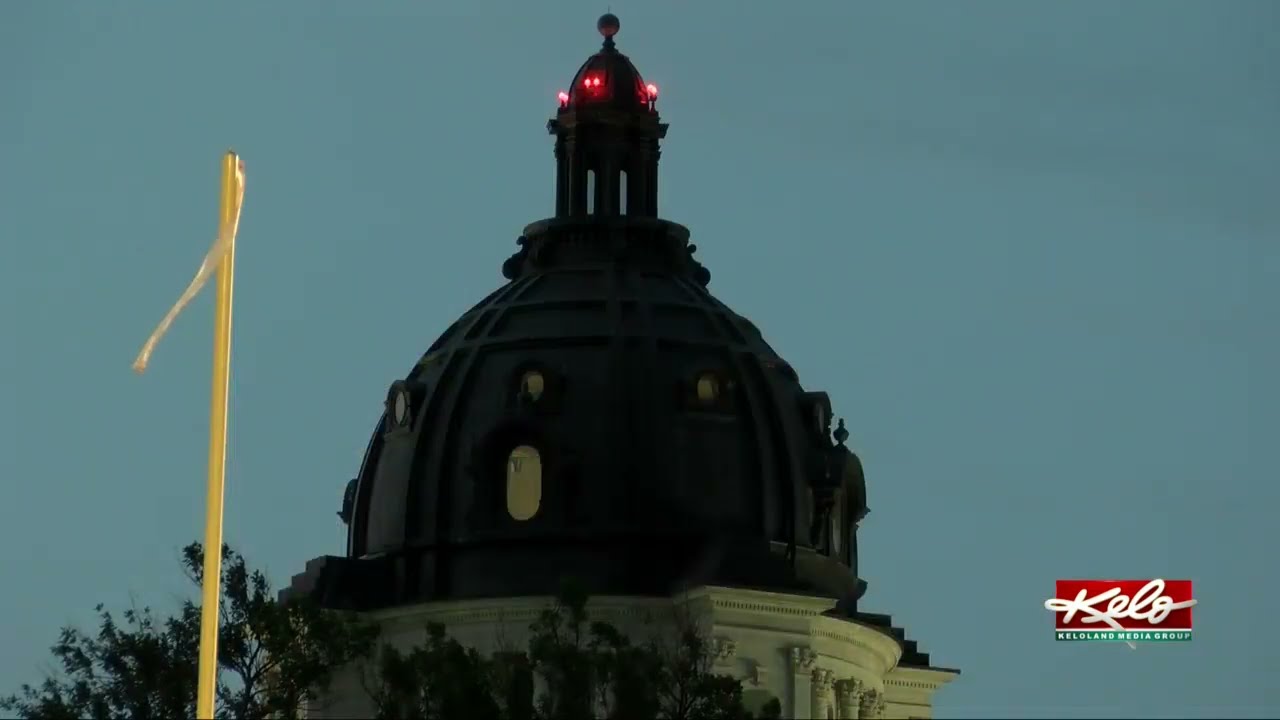The image is an exterior photograph taken at dusk, capturing the top of a domed governmental building. The dome is composed of a dark gray or black stone material, shadowy and adorned with red warning lights for aircraft. The building's lower portion is white, featuring columns and elaborate design elements. Tall dark green trees surround the structure. On the left, a tall yellow pole stands, topped with a long piece of cloth or streamer rather than a flag. In the bottom right corner, the text “KELO Land Media Group” appears, with 'KELO' prominently displayed in white flowing script on a red background.